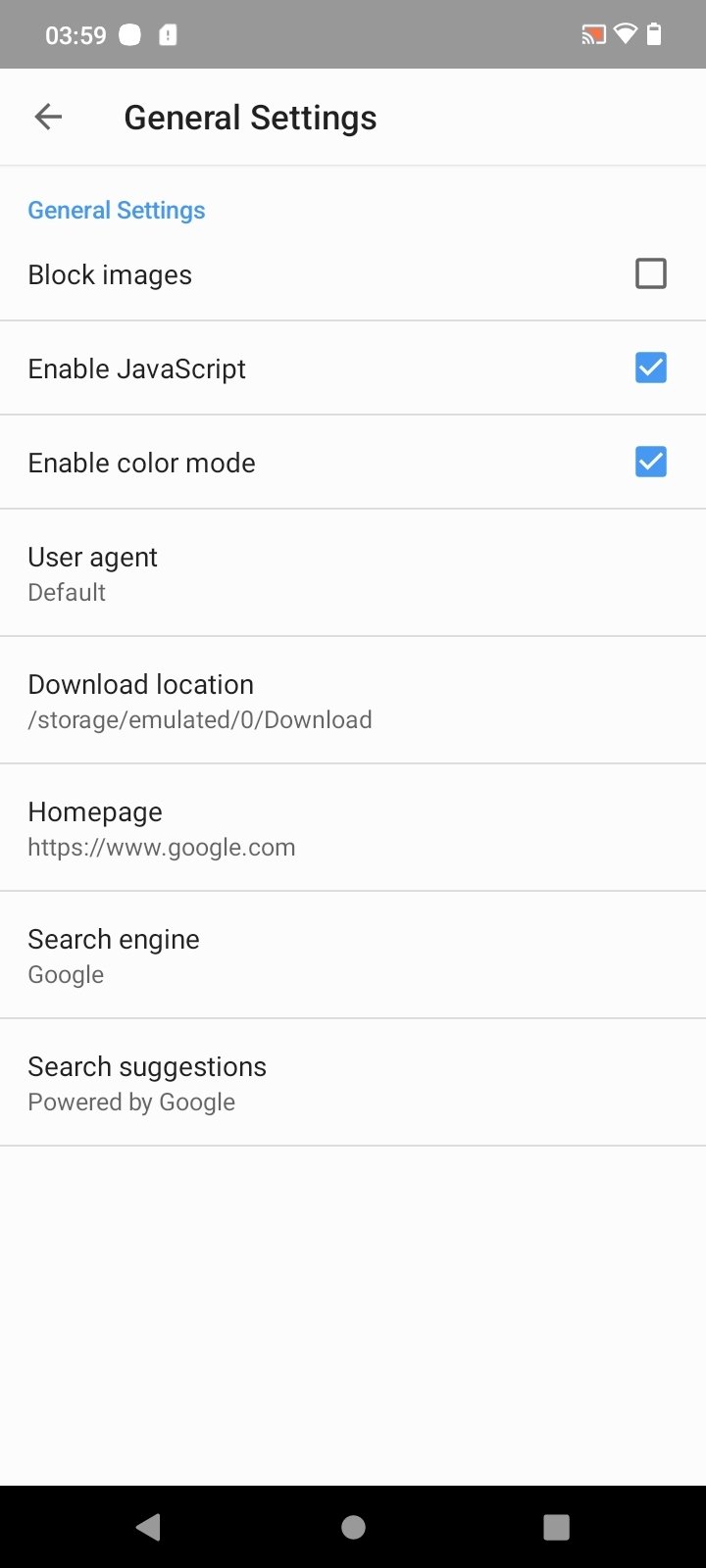A detailed screenshot of the settings page is shown. At the top, the page is titled "General Settings," accompanied by a back arrow icon on the left side. Each section is distinctly separated by horizontal lines, enhancing readability.

The first section includes "General Settings" in blue text on the left. Directly beneath it is the "Block Images" option, presented in black text, with an associated checkbox on the right side of the screen.

Following this is the "Enable JavaScript" option, which features a checked blue checkbox on the right, indicating that JavaScript is turned on. Continuing down, there is the "Enable Color Mode" option, also accompanied by a blue checkbox.

Further down, the settings list displays "User Agent Default," followed by "Download Location." The specific path for downloads is indicated as "/storage/emulated/0/Download."

Towards the bottom of the page, the "Homepage" setting is presented with the URL "https://www.google.com." Lastly, the "Search Engine" is set to "Google," and it is noted that "Search Suggestions" are powered by Google, with the URL "www.google.com" also mentioned.

The layout and options described suggest a comprehensive and user-friendly settings interface tailored for customization and ease of use.